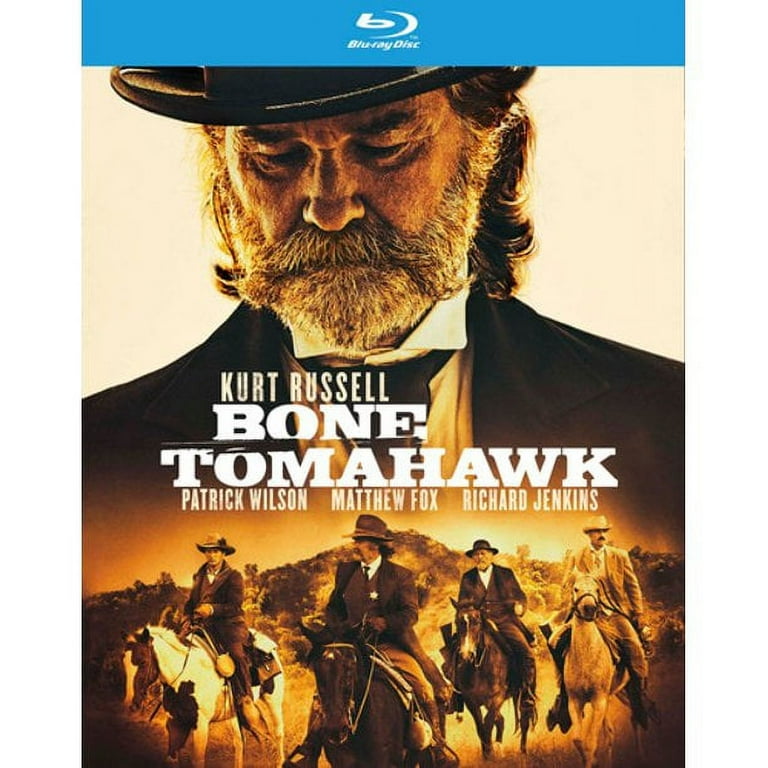The image depicts the cover of a Blu-ray disc for the movie "Bone Tomahawk." At the very top, a bright blue horizontal band prominently displays the Blu-ray logo. The central figure is a close-up of an actor with a rugged, straggly beard, thick sideburns, and shoulder-length wavy hair, dressed in an old-fashioned Western-style black suit, black tie, white shirt, and black hat. His deeply wrinkled face and downward glance add to the somber tone. Below this image, the names "Kurt Russell," "Bone Tomahawk," "Patrick Wilson," "Matthew Fox," and "Richard Jenkins" are listed. Further down, a lineup of four men on horseback, all wearing cowboy hats and suits, is showcased, with the central rider prominently featuring a sheriff's badge on his chest. The color palette of this lower part of the image consists of brown, cream, and white hues, emphasizing the Western theme.